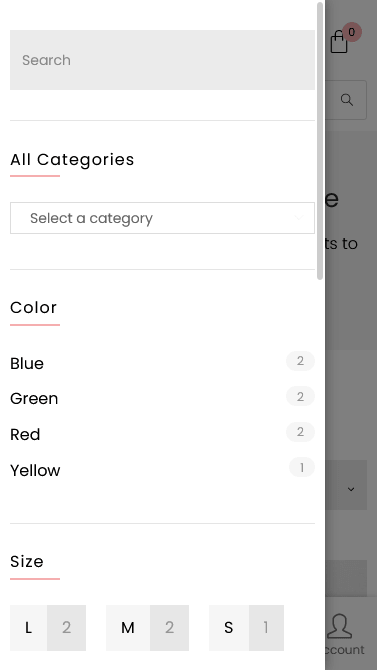This image features a screenshot set against a predominantly white background with various interface elements. At the top, there is a horizontal gray search bar that prominently displays the text "Search Inside." Directly below the search bar, the phrase "All Categories" is displayed in black text and is underlined with a red line. Below this, a boxed area contains the text "Select a Category." Further down, in bold red text, there is a heading for the color options, also underlined in red. 

The color options are listed vertically, each associated with a numerical value to the right:
- **Blue** (with a "2" to the right)
- **Green** (with a "2" to the right)
- **Red** (with a "2" to the right)
- **Yellow** (with a "1" to the right)

At the bottom of the screenshot, bold text reading "Size" is underlined with a red line. The available size options are arranged horizontally from left to right as: "Large," "Medium," and "Small."